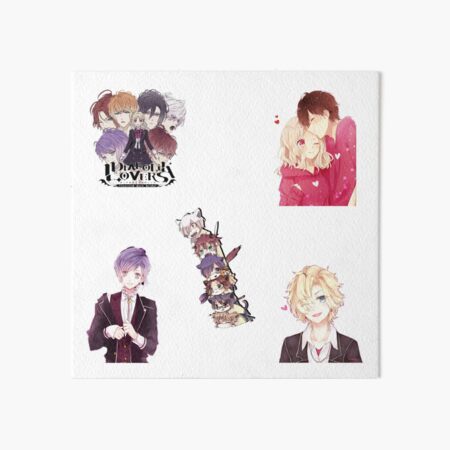The image shows a square piece of white paper divided into five sections, each depicting different anime-style drawings. 

In the upper left-hand corner, there's a panel with six heads of characters with short shaggy hair around a girl standing in the middle, dressed in a black outfit. The caption appears to say something like "Davy of the Varus" or "something Lovers."

In the upper right-hand corner, a girl with shoulder-length brown hair in a pink sweatshirt with a heart on it stands next to a man, also wearing a pink heart-decorated sweatshirt, with his head leaning towards her.

The lower left section features a woman with short purplish hair in a black jacket.

In the center section, there is a playful array of cats positioned as if on a sled, stacked in a totem pole-like manner.

The lower right corner shows a girl with wild blonde hair covering her eyes, wearing a brown jacket and a white shirt.

The drawing style looks like marker or watercolor, and the overall presentation has a distinct, vibrant anime flair.